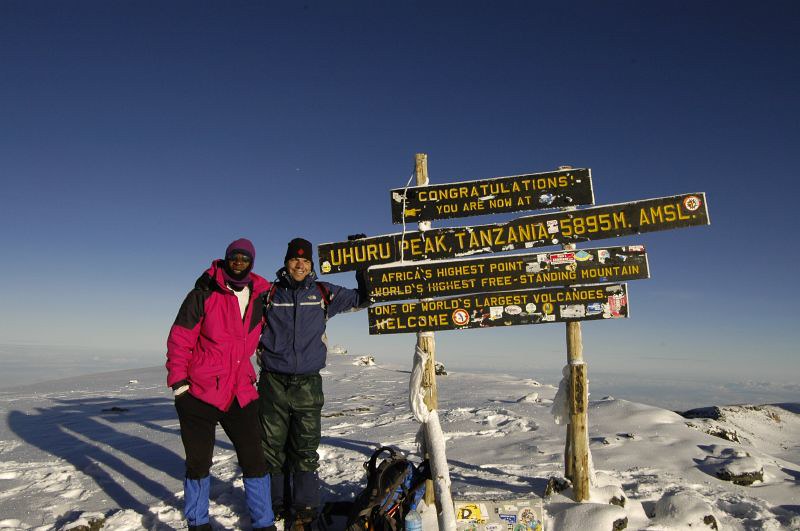The photograph captures a stunning outdoor scene of two men standing triumphantly at the snowy summit of Uhuru Peak, Tanzania, the highest point in Africa. The landscape is a striking contrast of crisp white snow blanketing the mountaintop and a clear blue sky above, which transitions from dark blue to light blue near the horizon. The two climbers, appearing accomplished and smiling, are dressed warmly in snow gear. The man on the left, who appears to be African American, wears a pink (or red) coat and black pants, while the man on the right, who appears to be Caucasian, sports a blue jacket and dark green pants. Both have caps to shield against the windy conditions. Behind them is a prominent wooden sign supported by two snow-buried posts, partially covered with stickers placed by previous hikers. The legible text on the sign reads: “Congratulations, you are now at Uhuru Peak, Tanzania, 5,895 M AMSL, Africa’s highest point, world’s highest freestanding mountain, one of the world’s largest volcanoes. Welcome.” Below the sign rests a backpack on the snow, and one of the men holds onto the sign for support. Their shadows, along with that of the sign, stretch behind them, reinforcing the clear and bright atmosphere of this high alpine achievement.